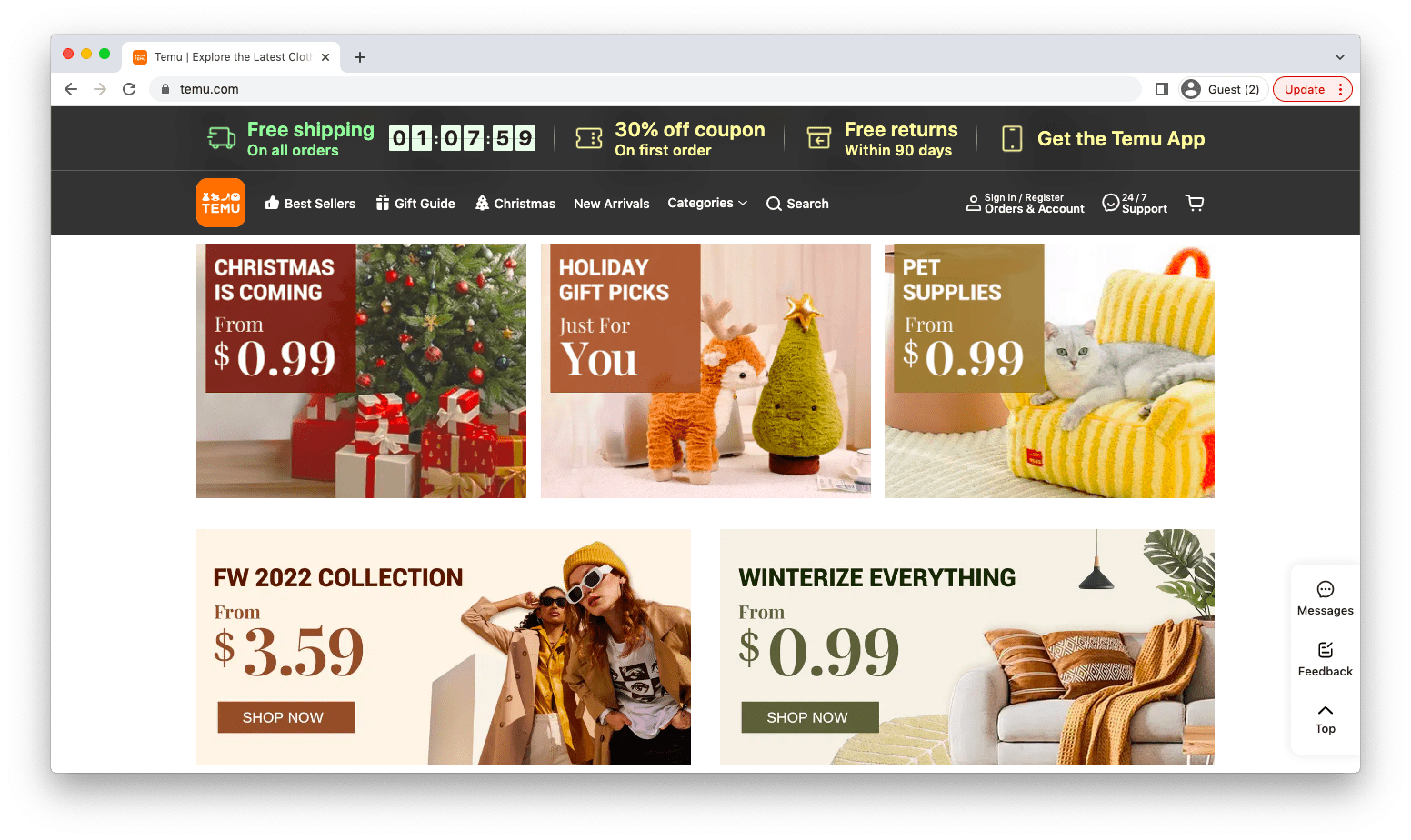The image displays the home page of TMU.com on an iOS device using the Google browser, as indicated by the guest profile and update notification. The address bar and browser tab both show "TMU.com." The website header reads "TMU - Explore the latest," inviting users to discover new products. 

Prominent advertisements dominate the front page. A banner announces "Christmas is coming," promoting holiday items starting at 99 cents. Another ad features a variety of holiday gift packs, including ornaments and other festive items. The pet supplies section, also starting at 99 cents, is illustrated with an image of a cat on a cat bed. A "Winterize Everything" banner suggests products like blankets, starting from 99 cents. Additionally, the FW 2022 Collection is advertised with prices starting at $3.59, showcasing stylish clothing modeled by two women, implying a women's fashion collection.